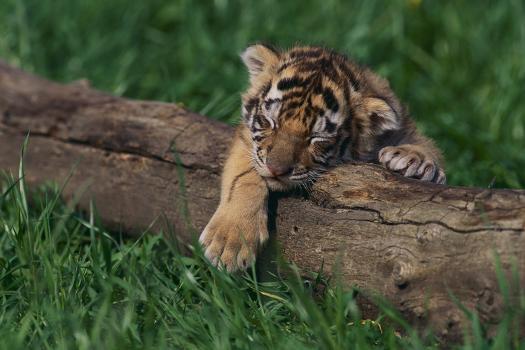In this full-color professional photograph taken outdoors, a baby tiger, or tiger cub, is nestled atop a weathered brown log that stretches diagonally from the upper left to the lower right. The log, devoid of any bark or branches and deeply cracked from age, is positioned in a lush, green grassy field. The cub, resting peacefully with its eyes closed and ears down, appears to be sound asleep. Its head is gently laid across the top of the log, and its left paw dangles over the side while the right paw rests back on the log. The tiger's fur, a mix of light orange, yellow, and brown with distinctive black stripes, also features white patches around its eyes and mouth, with a delicate pink nose adding to its charm. Shadows directly beneath the cub suggest it is the middle of the day. The serene scene conveys an image of tranquility and innocent repose.